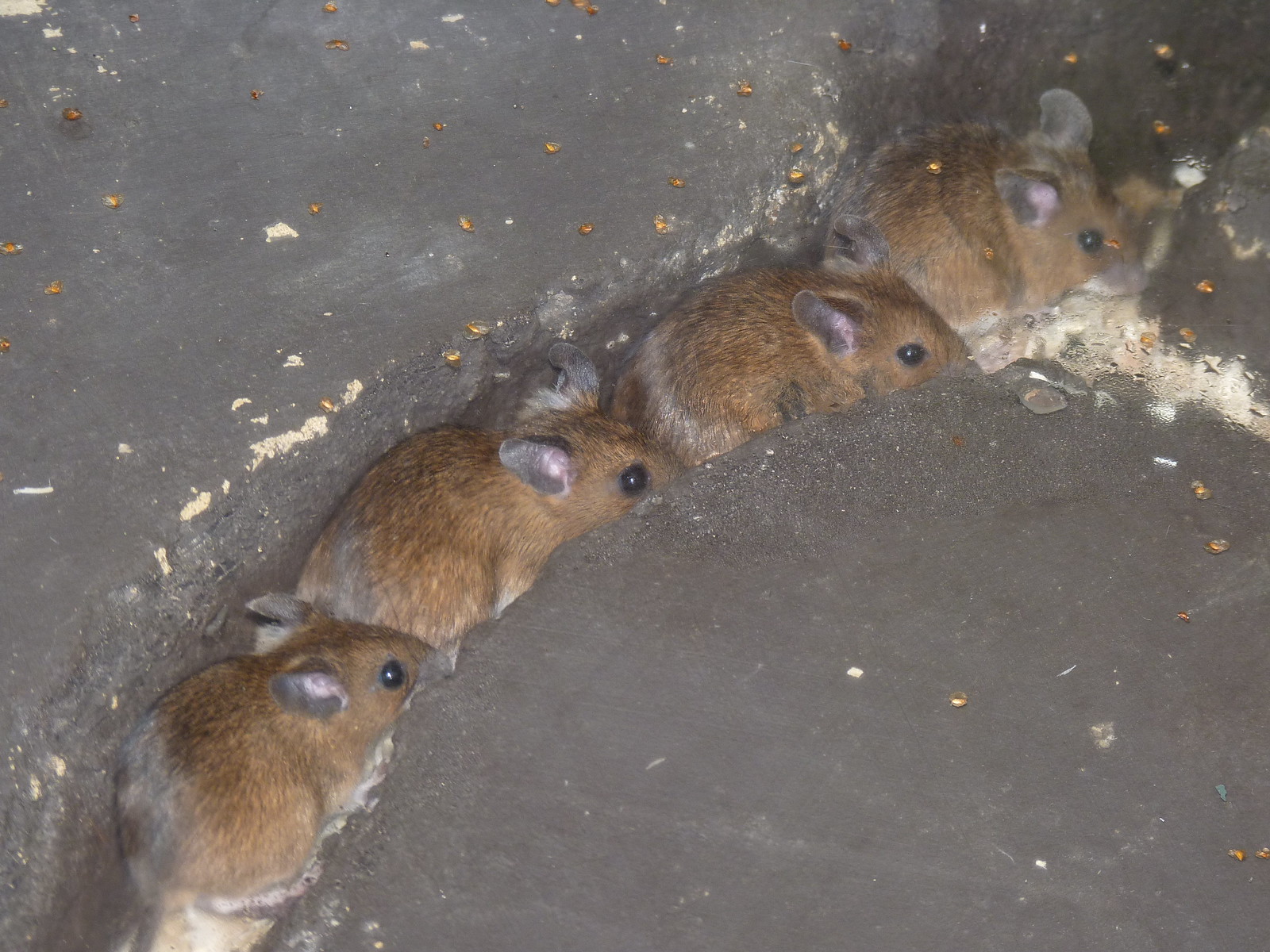This detailed photograph captures four small, brown mice nestled in a crack or groove within a stone or concrete surface. The mice, lined up head to tail, appear almost identical with their brownish fur marked by darker patches on their backs and big black eyes. Their ears are visibly large with a hint of pink inside. The ground they occupy is gray and stone-like, sprinkled with small grains or possibly bits of gold or flour, suggesting a setting that could be an outdoor sidewalk, a bakery, or a granary. The tight formation of the mice, coupled with their beady eyes and ear positioning, gives the impression they are either hiding or huddling together for warmth. The image has a close-up focus, limiting the view of their surrounding environment but emphasizing the texture of the stone floor and the mice's detailed features. The photographic clarity varies, with the mouse on the far right appearing slightly blurry, adding an intriguing depth to the composition.